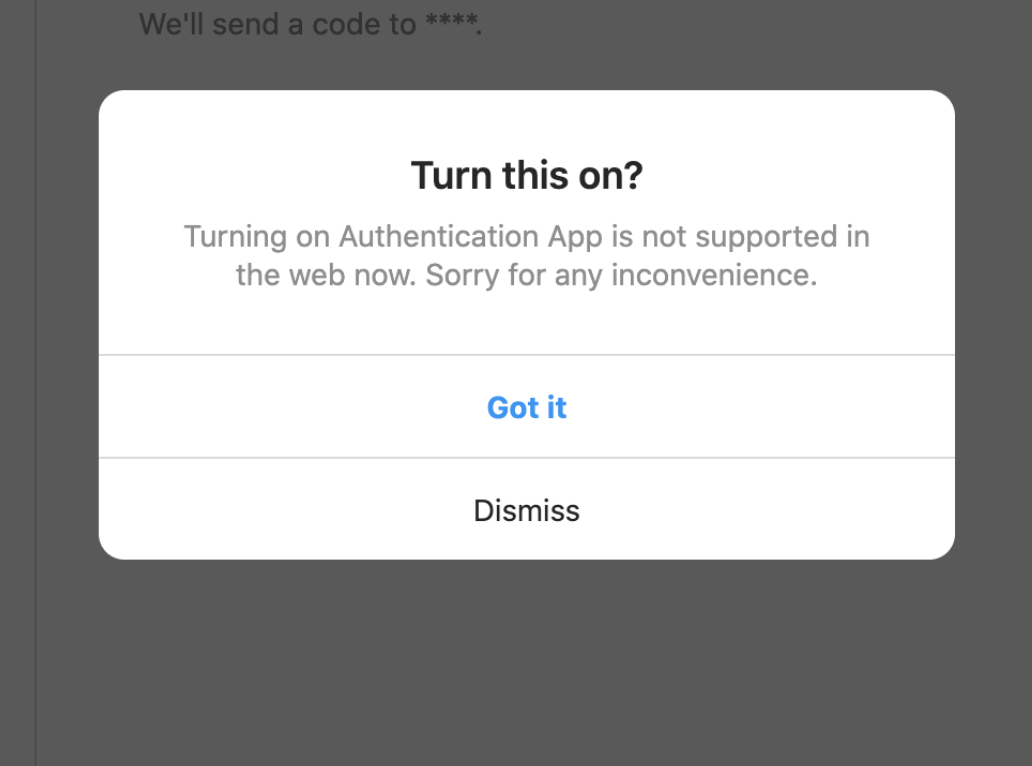In this image, there is a dialog box prominently displayed in the foreground. The dialog box contains a message that reads: "Turn this on. Turning on the authentication app is not supported in the web now. Sorry for any inconvenience." Below this message, there are options to acknowledge or dismiss the dialog with buttons labeled "Got it" and "Dismiss," and a "Close" button is also visible. The text within the dialog box is a mix of gray and blue colors, providing important instructions and feedback to the user. The background of the image is white, creating a stark contrast to make the text in the dialog box stand out more clearly.